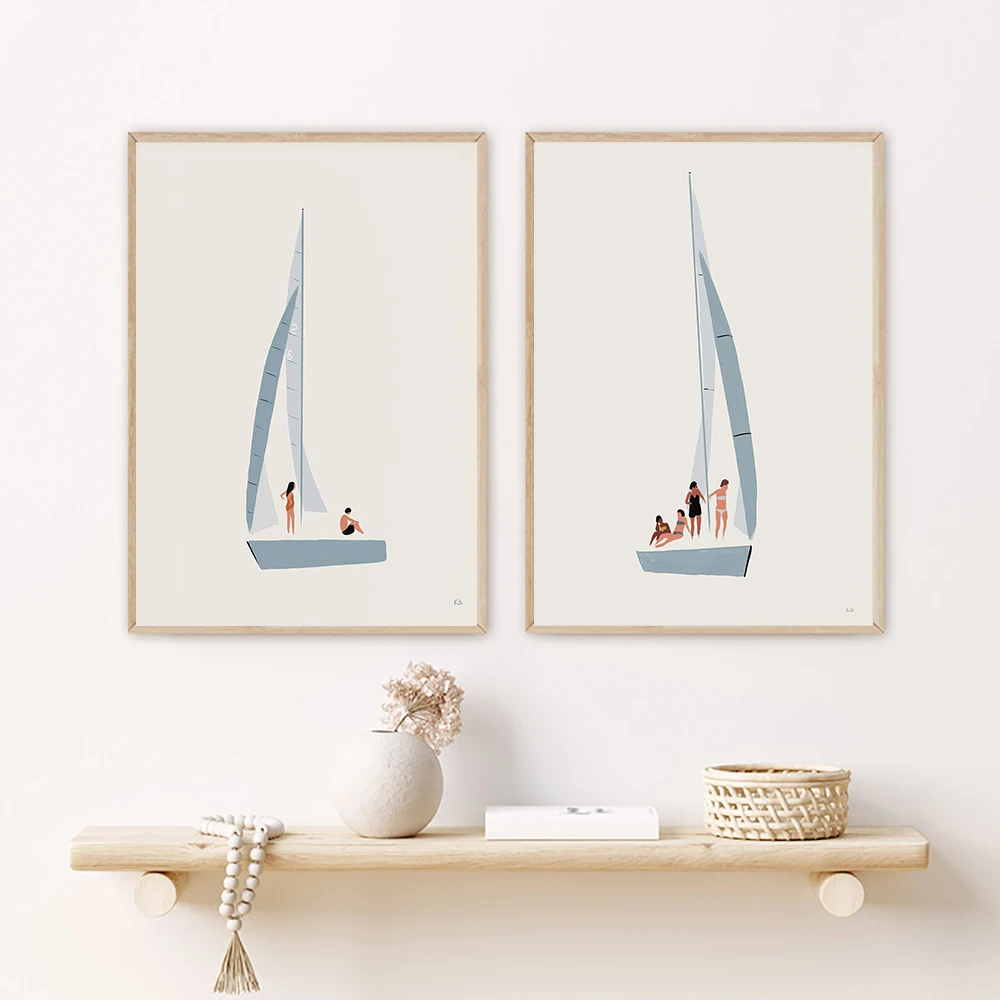This image features a wooden shelf mounted on a white wall. The shelf comprises a flat wooden board supported by two circular wooden brackets, suggesting the board is simply placed atop the brackets and can be easily removed. On top of the shelf, there is a white circular vase containing flowers, positioned next to a beaded necklace. To the right of the vase, there is a small wicker basket, and a book is situated between the vase and the basket. Above the shelf, the white wall showcases two framed pictures of sailboats in light wooden frames. The painting on the left depicts a gray sailboat with white, dark gray, and light gray sails, featuring a man in black swim trunks sitting on the boat and a woman in a red bikini standing nearby. The painting on the right shows the same colored sailboat with four women on it—two standing and two sitting. The sailboats in both paintings are similar in style and color, with the one on the left having two occupants and the one on the right having four.